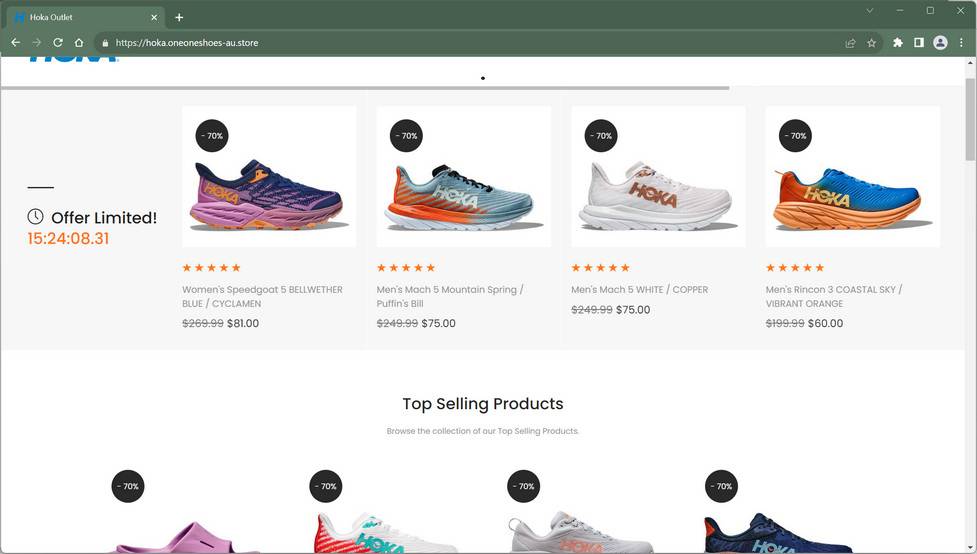This image showcases a promotional webpage from Hoka Outlet featuring a collection of discounted shoes. The webpage header includes navigation options such as forward, back, refresh, and home, indicating a user-friendly interface for shoppers. The web address displayed is https://hoka.onesshoes-au.store.

Beneath the header, the page is segmented into two rows of product images. The top row includes four pairs of shoes, each prominently labeled with significant discounts.

1. **Women's Speed Goat 5 Bellwether Blue / Cymaline**: Originally priced at $269.99, now available for $81, offering a 70% discount. The shoe features a striking purple and black color scheme with the Hoka logo on the side.
   
2. **Men's Mach 5 Mountain Spring / Puffin Bill**: Originally $249.99, now listed at $75, also with a 70% discount. This shoe is highlighted with a five-star rating and the Hoka branding on the side.

3. **Men's Mach 5 White / Copper**: Similarly discounted from $249.99 to $75, maintaining the 70% off deal and a five-star rating. This model is all white with copper accents, featuring the Hoka logo.

4. **Men's Rincon 3 Coastal Sky / Vibrant Orange**: Reduced from $199 to $68, with a 70% discount and a five-star rating, showcasing a vibrant mix of sky blue and orange hues, marked with the Hoka brand.

To the left side of the webpage, a notification highlights a limited-time offer ending in "15-20-4-08-31" (days, hours, minutes, seconds), urging customers to make quick purchasing decisions.

Below the top row, four additional shoes are displayed in another row, also marked with substantial discounts:
- A shoe with a purple upper.
- A white shoe with red accents on the back.
- A light grey shoe.
- A darker black shoe with teal Hoka branding.

At the bottom of the webpage, there are navigation options to browse the collection of top-selling products, with a scroll bar on the right for easy browsing.

The overall layout and detailed descriptions contribute to an enticing shopping experience, highlighting the significant discounts and variety of styles available in the Hoka Outlet promotion.